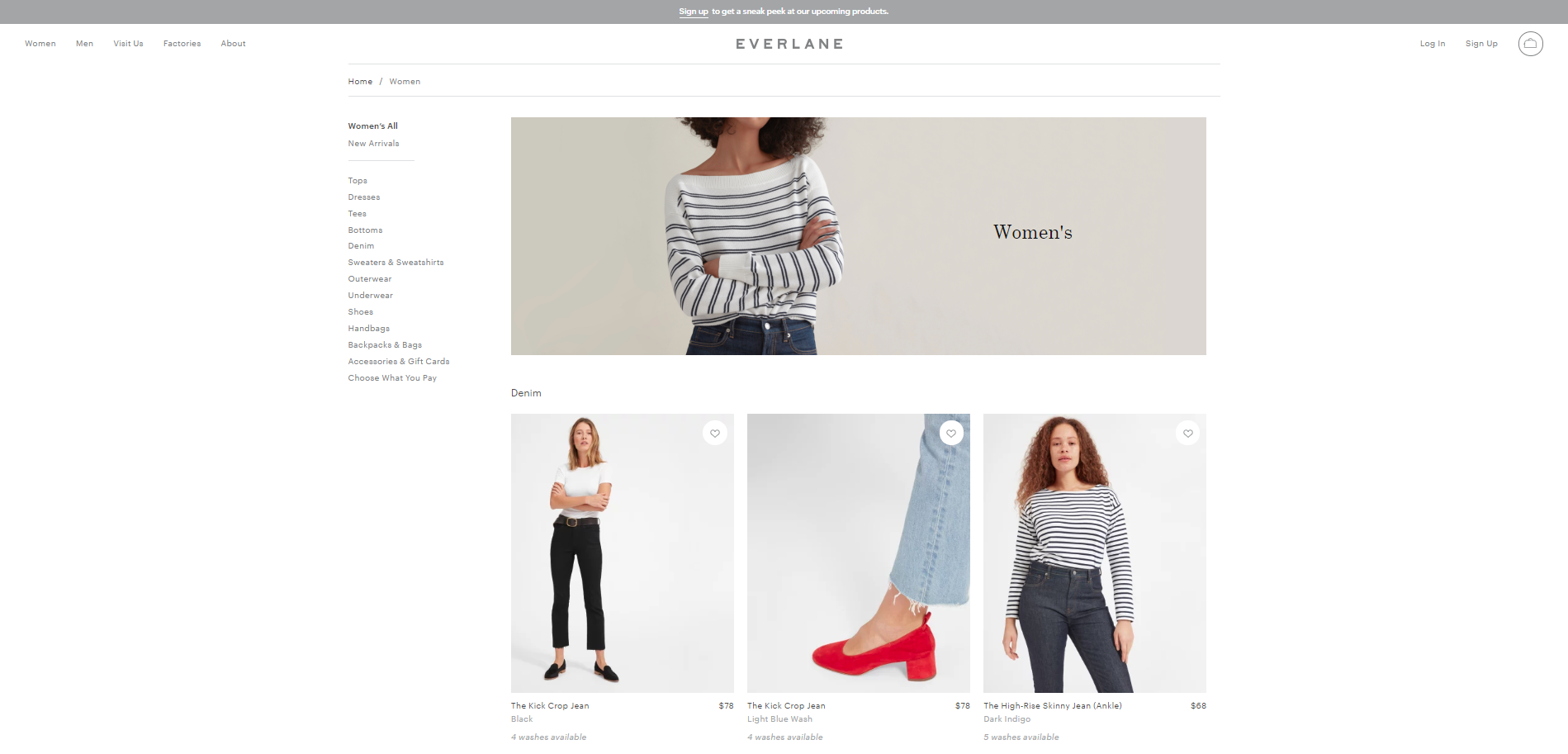The website for Everlane features a sleek design with a large yet thin gray banner spanning the top, adorned with minuscule text that's hard to decipher. Beneath this banner, there are navigational categories including "Women," "Men," "Visit Us," "Favorites," and "About," along with options to log in or sign up for an account.

The "Women" section is currently selected, indicated by a prominent image of a woman dressed in a long-sleeved shirt and jeans, accompanied by the label "Women" in an unimpressive, non-bold font. Below this image, there are various subcategories for women's clothing such as Tops, Dresses, and more, totaling around ten different sections.

Highlighted items in this section include:
- A woman without a visible face, showcasing a long-sleeved shirt and jeans.
- Another individual with arms crossed, wearing a plain white t-shirt, categorized under denim.
- A pair of jeans paired with regular shoes and no socks.
- A detailed shot of distressed denim paired with red shoes.
- A larger-sized model wearing a similarly striped shirt, possibly emphasizing size inclusivity.

Overall, the website's visual emphasis on the women's section reflects Everlane's collection of casual yet stylish apparel.